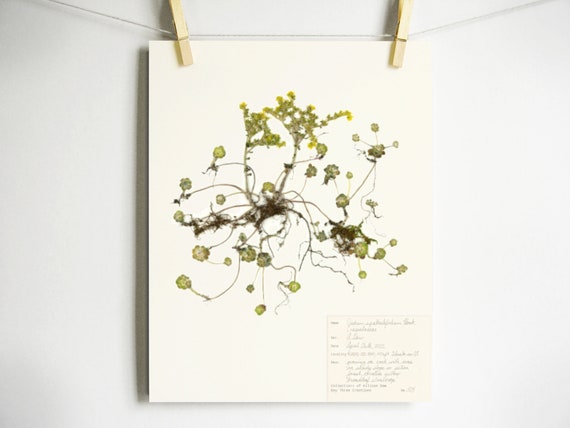The image is a color photograph displaying a piece of white cardstock with a color illustration of a plant, predominantly featuring green leaves and brown roots or branches, and possibly painted with watercolors. This cardstock is attached at the top by two light brown clothespins to a white string, which stretches across the image. The illustration appears to depict a plant with numerous thin tendrils and vegetation details. The background of the photograph is a plain white wall. In the bottom right-hand corner of the cardstock, there's a section of cursive script in black ink, though it is not legible. The photograph does not include any people, animals, or buildings, focusing solely on the illustrated plant against a minimalist backdrop.